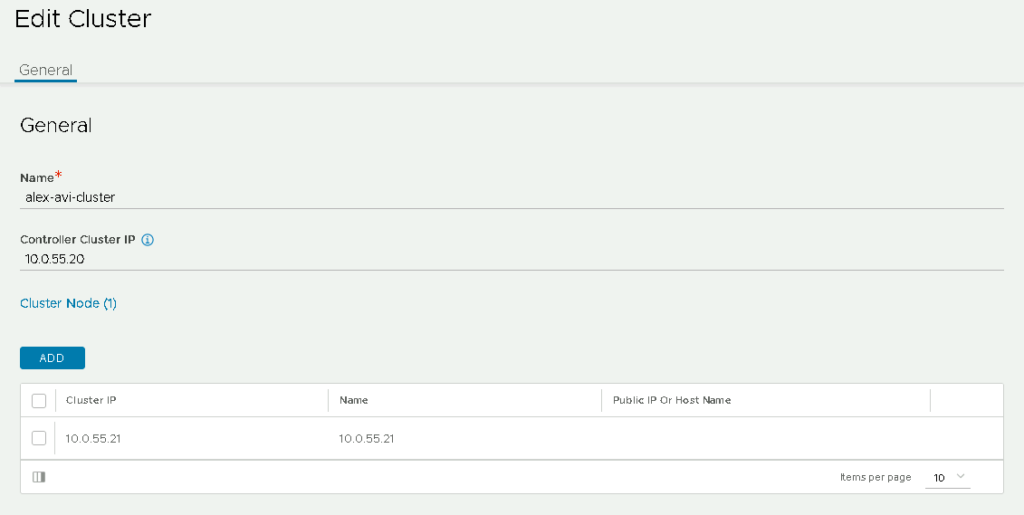This image is a cropped screenshot taken from a web page or a software application, depicting a user interface designed for editing cluster settings. The screenshot has a grey background and has been tightly cropped, excluding any web browser data or menu navigation options, showcasing only a specific section of the interface.

At the top, there is a prominent title labeled "Edit Cluster," followed by the word "General" twice, indicating the section's heading. Below this, the interface presents a text entry field labeled "Name" with a red asterisk, denoting a required field. Further down, there is another text entry field for entering a "Controlled Cluster IP," accompanied by a small icon of an eye within a circle, which likely serves as a toggle for viewing the IP address.

An option to add new clusters is highlighted in blue, inviting the user to expand the cluster list. Below these input fields, the existing clusters are organized in a white table with three columns: "Cluster IP," "Name," and "Public IP or Host Name." Currently, the table displays only a single cluster item, although the settings indicate that up to 10 items can be viewed per page. The table format ensures clarity and ease of data management, crucial for handling technical internet protocol information.